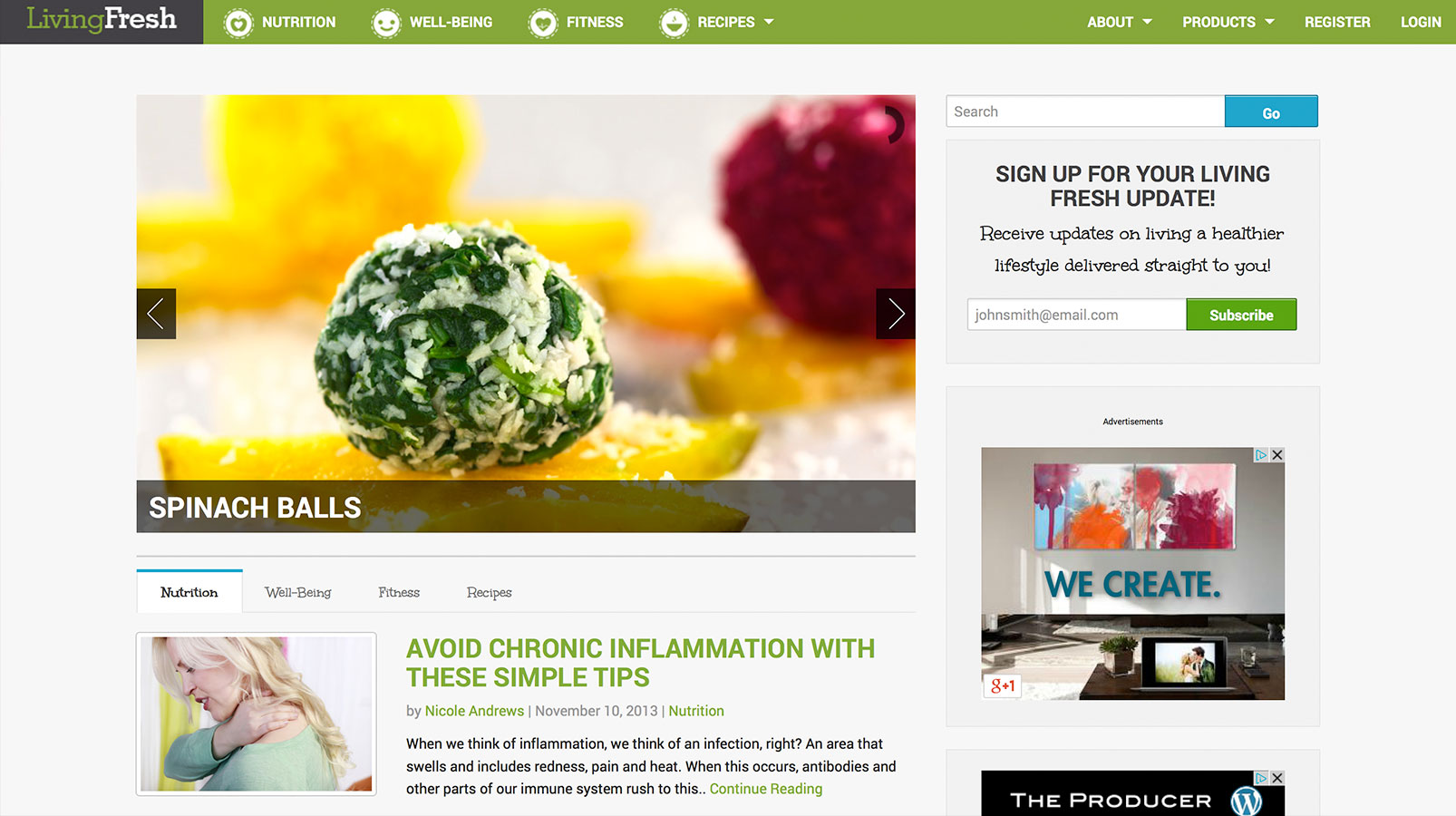**Website Screenshot: Living First**

The image showcases the homepage of a website named "Living First," with the logo prominently displayed on a black sidebar. The word "Living" is in green text while "First" is in white text.

At the top of the page, there's a green navigation bar featuring the following sections in white text: "Nutrition," "Wellbeing," "Fitness," and "Recipes," each accompanied by relevant icons to the left. An arrow points towards the "Recipes" section, indicating it might be currently selected. On the right side of the navigation bar, additional options include "About," "Products," "Register," and "Marketing," all in white text.

The background of the page below the navigation bar transitions to white with light gray accents. Central to the page is the heading "Spinach Bowls," likely indicating a specific recipe page. Below this heading is a horizontal bar with white text, and a small image of a spinach bowl sits atop a yellow bar, accented with a slice of fruit.

In the top right corner of the page is a search bar with a blue "Go" button beside it. Below the search bar, there's a call-to-action message encouraging users to sign up for "Living Fresh" updates, emphasizing the benefits of staying updated on health and wellness. This message is accentuated with an exclamation point and employs a more casual Comic Sans font, contrasting with the professional capitals above it. 

To the side, there's an ad that appears similar to a Google ad, featuring the word "Recreate" and another text reading "Khabar" in the room. Underneath the spinach bowl image, additional sections focus on "Nutrition," "Wellbeing," and "Fitness." The "Nutrition" section highlights an article titled "Avoid Chronic Inflammation with These Simple Tips," accompanied by an image of a woman holding her shoulder.

The combined visual elements and text indicate an organized, health-focused website aimed at providing valuable information and recipes to its users.